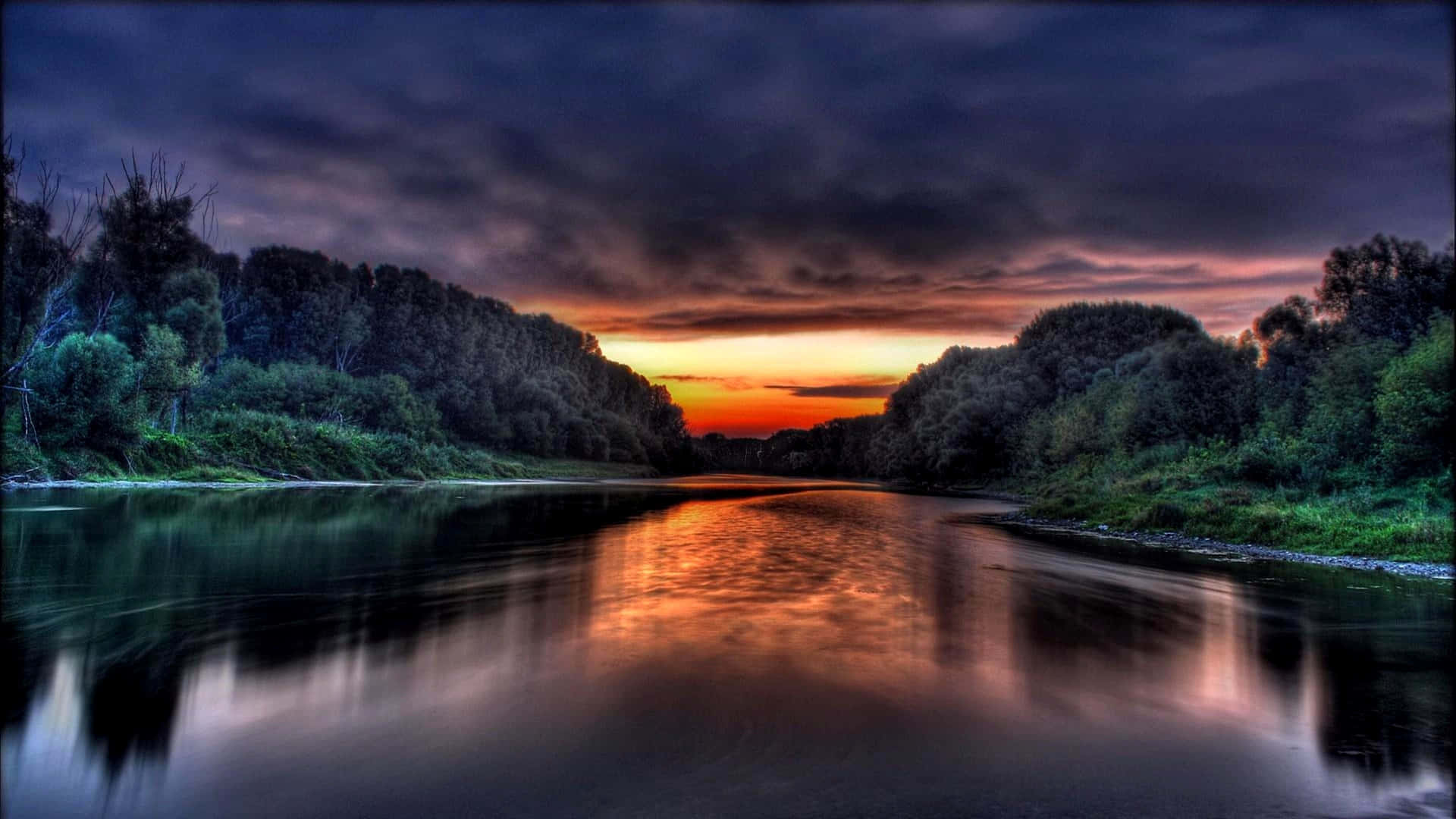The image portrays a stunning sunset over a tranquil waterway, possibly a lake or river, with a digitally enhanced appearance. Central to the scene is the serene water reflecting the sky's dramatic colors, ranging from deep black at the top to vibrant yellow and orange hues towards the horizon, where the sun is setting low. Dark, brooding clouds dominate the upper section, gradually giving way to a clearer, lighter distance. Lush greenery lines both sides of the water, with trees, bushes, and grass transitioning from vibrant green in the foreground to darker greens and blacks further away, adding depth to the scenery. Silhouetted trees in the far distance, combined with the slight mist and reflective quality of the water, enhance the surreal, almost magical atmosphere of the landscape.